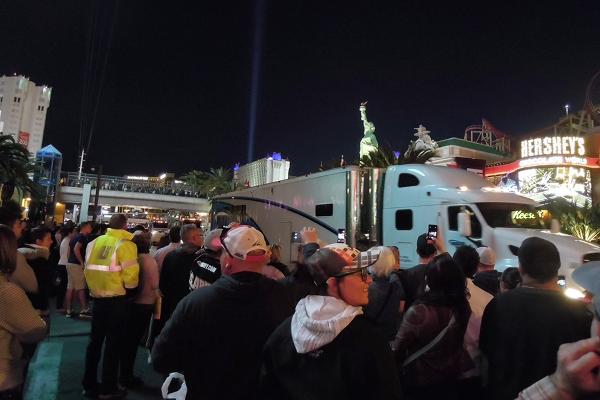The image captures a bustling nighttime scene, likely in Las Vegas, with a crowd gathered on a sidewalk. In front of the crowd, a large white semi-truck, possibly a food truck, is present. On the right side of the frame, there's a brightly illuminated sign reading "Hershey's Chocolate World," indicating the presence of the famous chocolate company. In the distance behind the truck, a model of the Statue of Liberty stands out against the dark sky. To the far right, the backdrop includes a possible roller coaster or other amusement structures, hinting at a recreational park. On the left side of the image, a tall, many-storied white building rises, adjacent to a walkable bridge crowded with people. Additionally, a beam of blue light extends skyward from a rectangular building located left of the Statue of Liberty replica. The scene is vibrant and energetic, with numerous people milling about, absorbing the lively atmosphere of what appears to be a significant event in an entertainment-centric location.